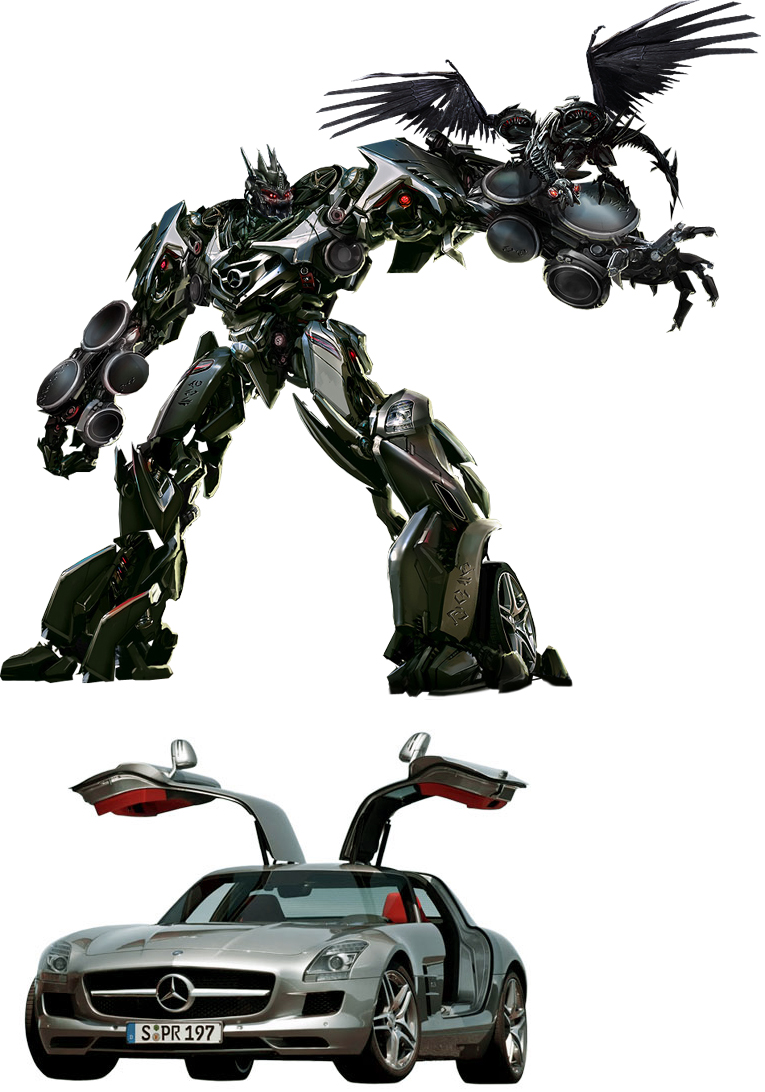The image consists of two distinct parts displayed against a white background. The top portion features a highly stylized, computer-generated metallic robot that resembles a character from the Transformers series, specifically a Decepticon. The robot, assembled from various spare parts, has two legs, two arms, and numerous black circular plates on its body. It sports a pair of black wings on its left arm, and its head is adorned with prominent spikes. A black robotic bird is perched on its left arm, adding to its intricate design. The bottom portion of the image displays a massive, vintage silver sports car, identifiable as a Mercedes-Benz with the distinctive gullwing doors that open upwards. The car features a white license plate with the number SPR197 in black letters. The curved shape and upward-opening doors of the car are reminiscent of classic models like the DeLorean.